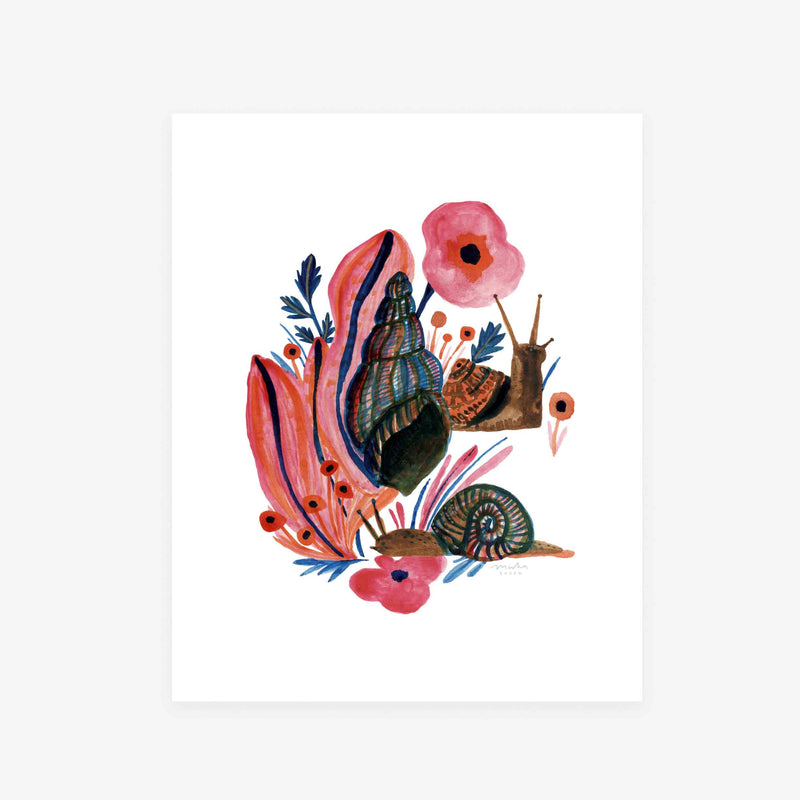The image depicts a vibrant, watercolor-style scene set against a white background, featuring two brown-bodied snails with varied, dusty-colored shells in shades of brown, red, blue, and tan. The snail in the lower part of the composition is crawling along the ground, with an orange and blue patterned shell, while the snail above it stands erect with an orange and brown-patterned shell and its antennae pointing straight up. To the right of the standing snail is a large, multicolored seashell with a dusty blend of blue, red, and tan hues. The background is adorned with clusters of vivid pink flowers, including one prominent large flower and several smaller ones, interspersed with orange flowers and deep blue-green leaves. Red seaweed and other seagrass add an unexpected pop of color, creating a whimsical underwater landscape. The artist's signature is visible beneath the crawling snail, grounding the ornate composition in a signature style that combines the fantastical elements with natural underwater themes.